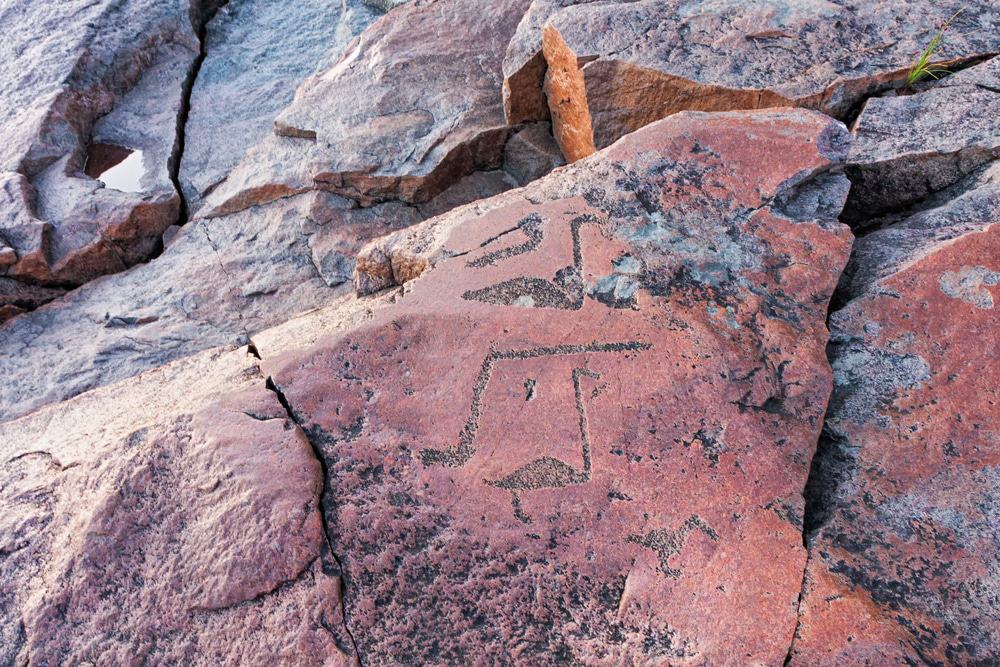This is a detailed outdoor photograph capturing a striking rock formation dominated by reddish-orange and grayish tones. The rock face features distinct jagged and flat surfaces, with numerous cracks and straight edges contributing to its rugged appearance. In the upper left-hand corner of the image, a small pool of water is visible, and in the upper right-hand corner, a small green plant adds a touch of life to the scene. Notably, one of the prominent rocks has a hole through which a sliver of sky can be seen, and this rock, along with others in the foreground, contains various etchings that resemble hieroglyphics. Among these etchings are shapes that look like birds, swans, and ducks, suggesting they might not be naturally occurring. This rock formation, with its intriguing carvings and natural elements, forms a visually compelling and multi-faceted landscape.